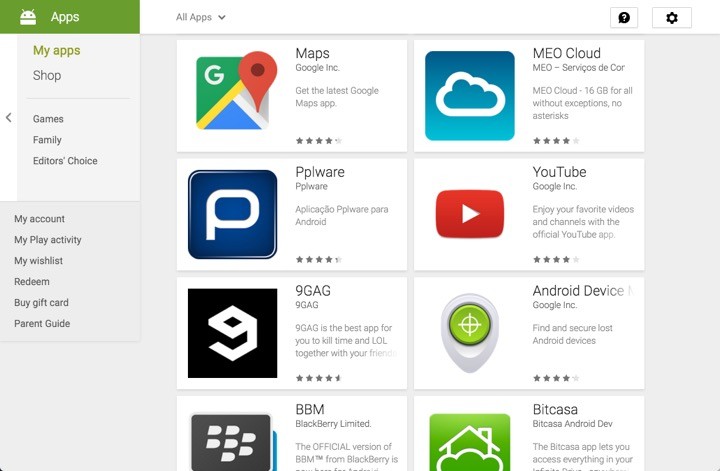The image is a screenshot of someone's app management page. 

At the top left corner, there is a small icon resembling an alien or bug. Next to this icon, there's a green rectangle with the word "Apps" written inside. Below this section, the options "My Apps" and "Shop" are displayed. Further down, there are additional categories listed: Games, Family, Editor's Choice, My Account, My Play Activity, My Wishlist, Redeem, Buy Gift Card, and Parent Guide.

Centralized at the top, the header reads "All Apps," organized into two columns with four apps each. The left column lists the apps as follows: 
1. Maps (by Google Incorporated)
2. PPLware
3. 9GAG
4. BBM

The right column lists the apps as follows:
1. MEO Cloud
2. YouTube (by Google Incorporated)
3. Android Device
4. Bitcase

At the top right corner, there is a speech bubble with a question mark inside, and a settings gear icon enclosed in a square.